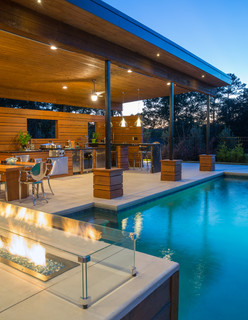The image depicts a serene twilight scene in someone's backyard, featuring a built-in swimming pool partially visible on the right. The pool's blue water reflects the sky and the supporting posts of a luxurious outdoor seating area. To the left, there's a spacious structure with a ceiling of brown wood and embedded lights, supported by posts with stanchions that appear to be either cement or wood. This open area has a gray cement floor and includes several amenities: a table, possibly with a TV mounted on the wooden wall behind it, a partial view of a metal chair and table, and an intriguing feature resembling a cooler or bar area with a brown wood exterior and a white Formica-like top covered with plastic. Additionally, there is mention of a banquet serving table with a cover, and some patio chairs, potentially beach chairs, nearby. The scene is framed by a backdrop of trees and, though it is twilight, the sky maintains its blue hue with a whitish glow on the right from the setting sun. There also seems to be an intriguing element—a low fire feature encased in glass, resting on some rocks, providing a focal point reminiscent of outdoor restaurant settings.